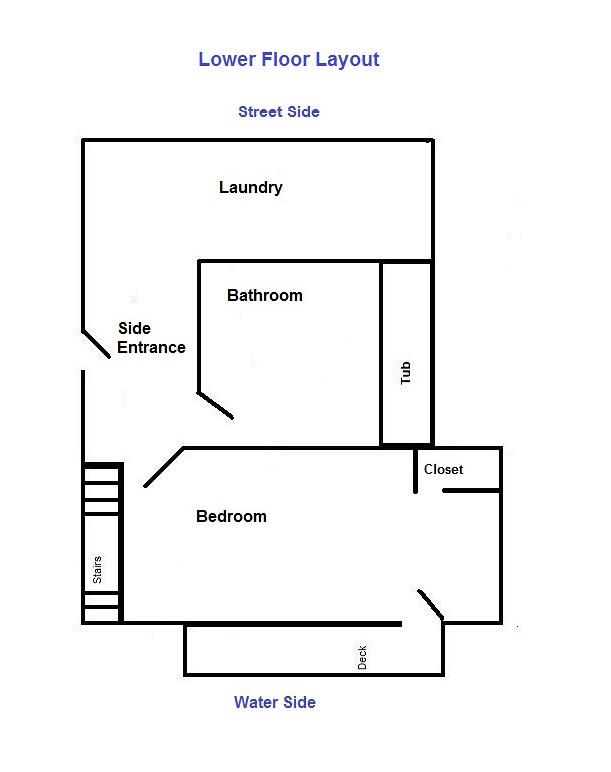This image showcases the blueprints for the lower floor layout of a house, with detailed labels indicating specific areas. Notably, the floor plan identifies the "Side Street" location, providing an orientation for the viewer. The layout features a spacious laundry room that includes a side entrance. Adjacent to this entrance is a bathroom, which is equipped with a tub. 

Moving through the layout, the blueprints reveal the presence of stairs leading to a bedroom. This bedroom includes a closet and offers access to a deck, which is notably labeled "Water Side" in navy blue lettering, suggesting the presence of a nearby body of water. Judging by the overall layout and design, the house appears to be a compact, yet efficiently designed beach house, potentially situated by a lake or ocean. The floor plan, while well-labeled and clearly indicating various sections, remains a rough and preliminary outline without images or detailed descriptions of the specific features within each room.